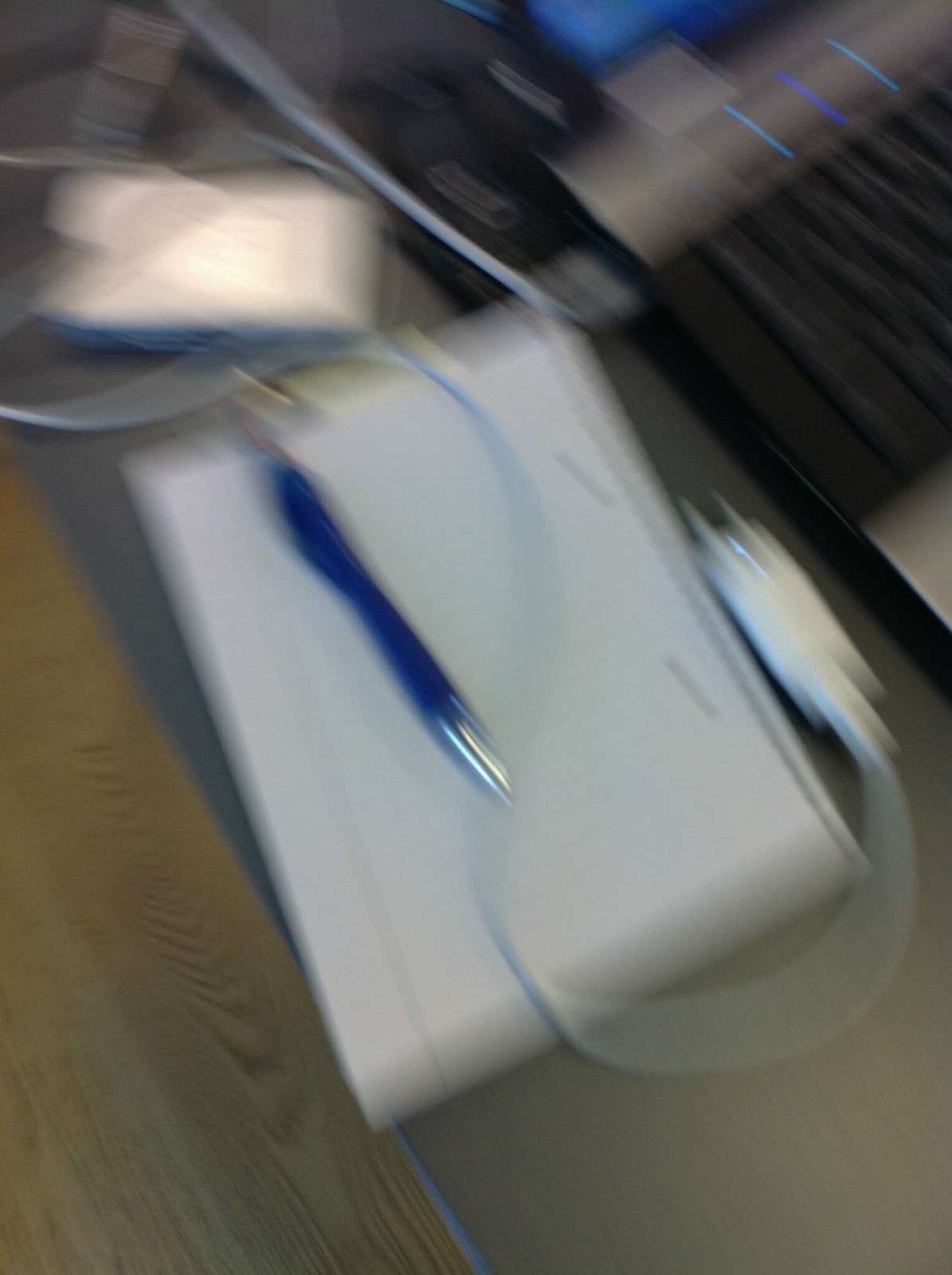This image, though blurry, captures a scene that hints at a casual workspace. In the lower left-hand corner of the picture, a wooden floor is visible. Nearby, there is what appears to be a gray table surface. Resting on this table is a notebook, identifiable by a spiral binding along its right edge. Atop the notebook, there is a blue pen with a silver tip. Additionally, a white cord, possibly a phone charger, meanders across the notebook, forming a shape reminiscent of a backward 'S,' with the plug extending off the side of the notebook.